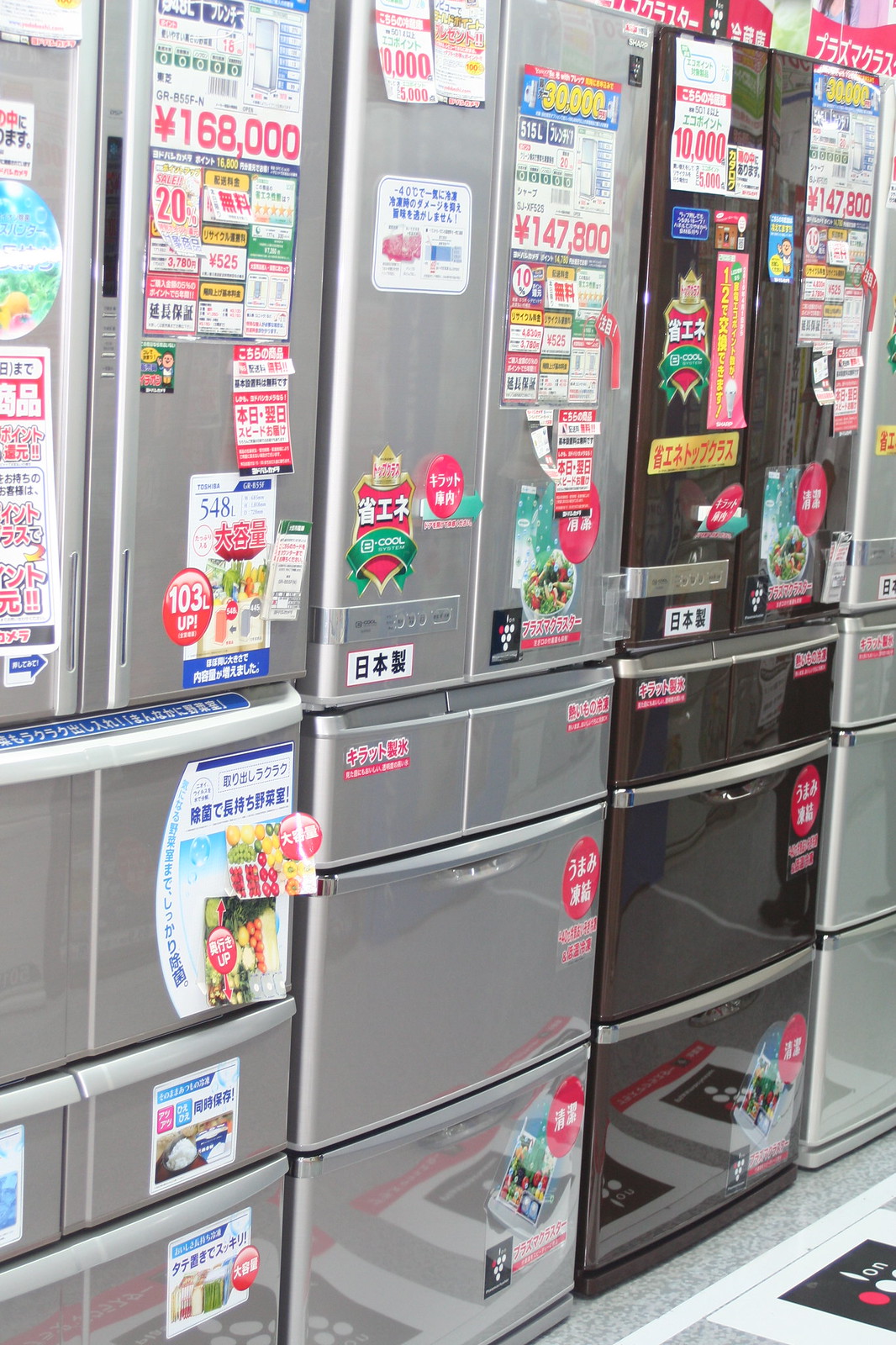The image depicts a row of refrigerators for sale in a store, viewed from an angle that makes the left side appear closer to the camera than the right side. The refrigerators are lined up against a back wall, with a light gray floor visible in front of them. The first refrigerator, on the left, is a gray stainless steel model featuring two top doors with gray handles, followed by a pull-out drawer beneath them. Below this drawer are two side-by-side pull-out drawers, and at the very bottom, a single pull-out drawer. The front of this refrigerator is covered with stickers displaying prices and sales information.

To the right of the first refrigerator is another stainless steel model with dark gray handles. It has double doors on top and three single pull-out drawers stacked below it. Like the first, this refrigerator is also adorned with numerous stickers and tags.

The last refrigerator on the right is black, with double doors on top and three pull-out drawers beneath. This appliance, too, is heavily decorated with price tags and informational stickers. The combination of foreign language labels and different currency symbols on the stickers suggests that this image might have been taken in a store outside of the United States.